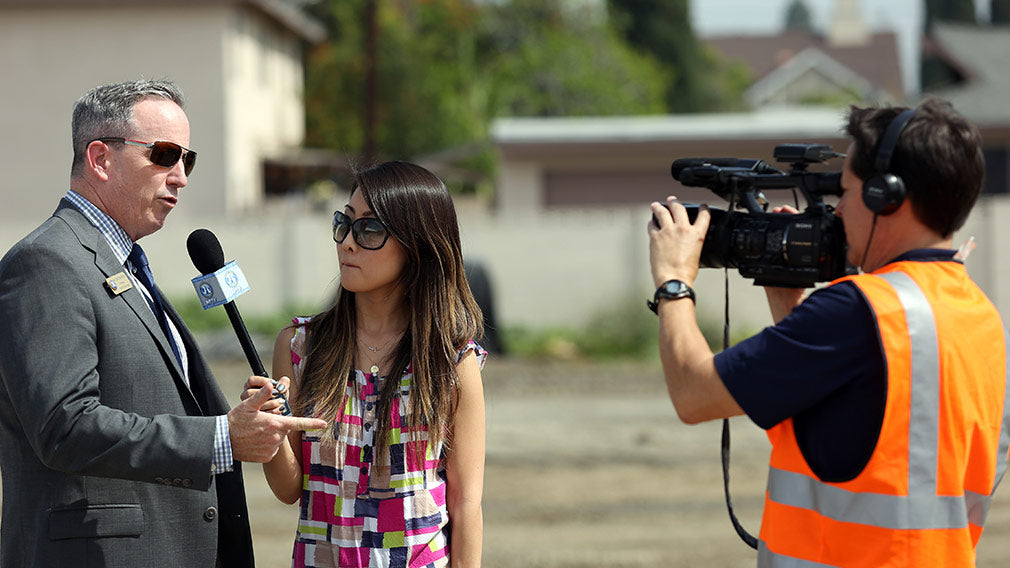In this detailed color photograph, a man is being interviewed by a woman on his right. The man, standing on the left side of the image, is dressed in a gray suit paired with a blue and white checkered shirt and a dark tie. He sports dark sunglasses and has short gray hair, with an unreadable name tag affixed to the lapel of his blazer. He is gesturing with one hand as he speaks. The woman beside him is holding a long microphone towards his mouth. She is wearing a sleeveless, multicolored square-patterned top and dark sunglasses, with long dark hair cascading over her shoulders. Facing the man, she listens attentively to his words.

On the right side of the image stands a cameraman documenting the interview. He is clad in a black shirt under a neon orange high-visibility vest with silver lines. Headphones cover his ears as he focuses on capturing the moment with his camera. The background features an out-of-focus white building with green trees visible behind it, indicating a serene, yet urban setting.